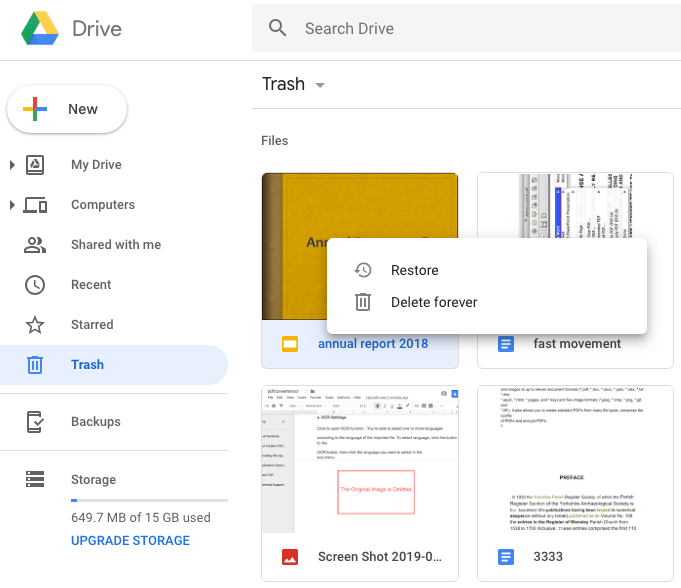The image displays a Google Drive interface, characterized by a clean, white background and a sleek, square design with gray labels. At the top, the familiar blue, green, and yellow Google Drive logo is accompanied by the word "Drive." Adjacent to the logo is a search bar labeled "Search Drive."

On the left side, a vertical toolbar includes various tabs: "New," "My Drive," "Computers," "Shared with Me," "Recent," "Starred," "Trash," and a "Backups" section. The "Trash" tab, highlighted in blue, indicates the current selection. Below these, a storage utilization bar reveals that 649.7 megabytes of the available 15 gigabytes are in use, with an "Upgrade Storage" button in blue situated nearby.

The main display area is dedicated to the contents of the "Trash" folder, which houses four files. Each file has options to "Restore" or "Delete Forever." The files listed include "Annual Report 2018," "Fast Movement," "Screenshot 2019," and a document titled "3333." The overall interface is seamless, providing an organized and intuitive user experience.